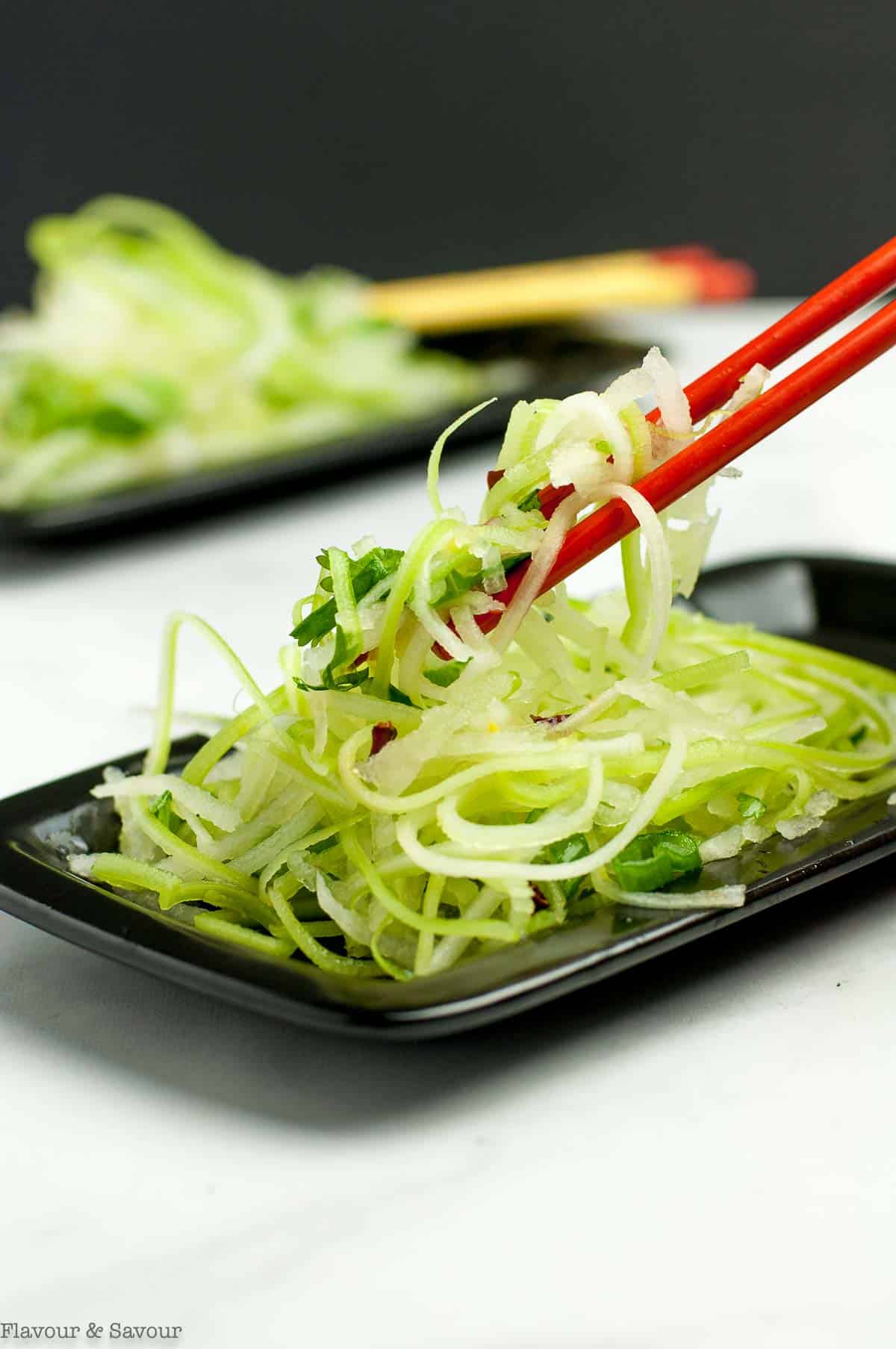The image showcases a detailed portrait-style photograph of a Japanese-inspired green vegetable salad, resembling zoodles or shredded lettuce, neatly arranged on two rectangular black plates with shallow middle sections. Set against a black background and placed on an off-white table, the focal point is the vibrant green salad being elegantly lifted by a pair of red chopsticks from the top-right corner. The stringy vegetables display a noodle-like form. In the background, another identical dish is slightly blurred, featuring green vegetables and a pair of yellow chopsticks with red tips positioned at the side of the plate, prepared for a second person. A subtle watermark at the bottom left corner reads "flavor and savor," enhancing the visual appeal of this meticulously composed culinary scene. The primary color palette includes shades of black, green, and red.